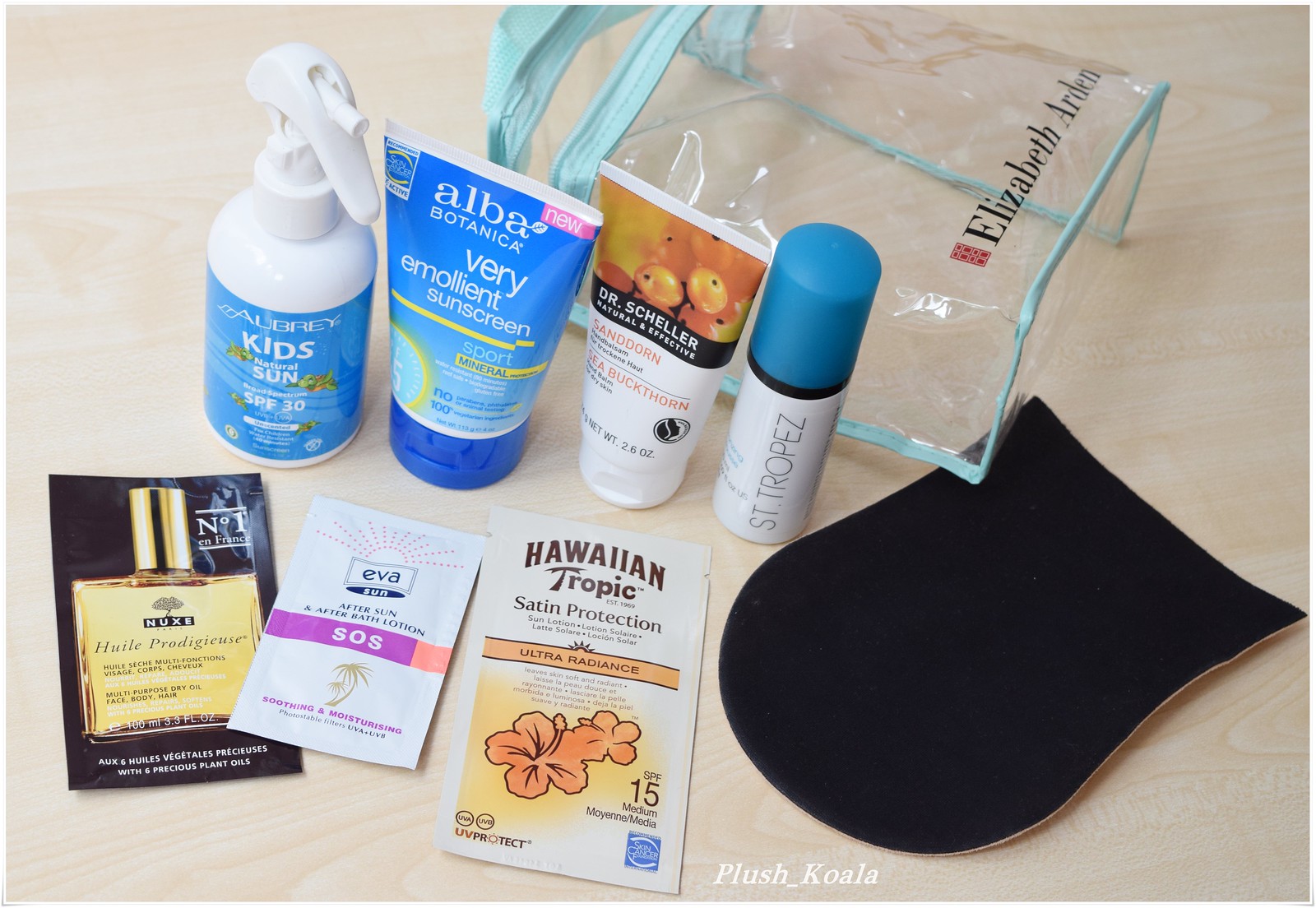The image depicts a neatly organized toiletries bag, apparently being packed for a trip. The bag itself is transparent with light blue or teal edges and features the brand name "Elizabeth Arden" emblazoned on the front. It has a zipper closure at the top. This compact and clear design indicates that it is suitable as a carry-on bag compliant with airline regulations for in-flight liquids. 

The bag contains various skincare products, each with specific attributes. Among them is a small spray bottle labeled "Kids Natural Sun SPF 30," designed for children's sun protection. Another notable item is a tube of "Alba Botanica Very Emollient Sunscreen," ideal for moisturizing skin while protecting it from the sun. Additionally, there's a tube labeled "Dr. Scheller Natural & Effective," which could be either a lotion or sunscreen. A smaller bottle reads "St. Tropez," likely containing a product from their self-tanning or skincare line. 

Several sample packets are also visible within the bag, including "No. 1 Perfume After Sun Lotion SOS Eva" and "Hawaiian Tropic Sunscreen SPF 15," both catering to after-sun care and additional sun protection. Among these items, there is also an enigmatic black, soft material item, the purpose of which is unclear from the current view.

All these items are meticulously placed on a light wood-colored surface, enhancing the visual appeal and neatly organized presentation of the travel toiletry essentials.